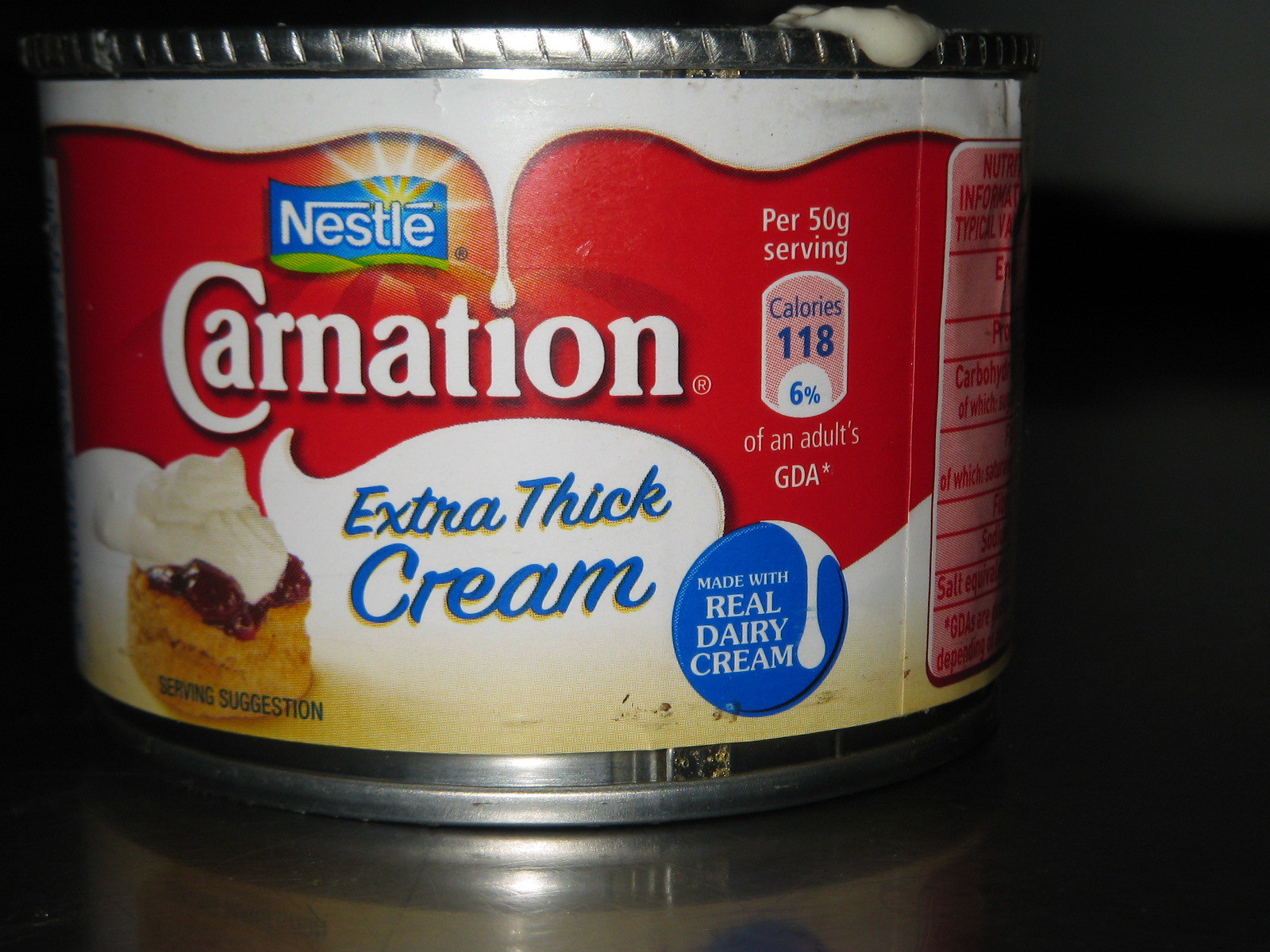In this image, a can of Nestle Carnation Extra Thick Cream is placed on a brown table against a dark gray wall. The can features a silver top with a small quantity of the cream spilling out. The label is predominantly white with a bold red band across the middle, interrupted by a small blue square with the Nestle logo in white letters. Above the logo, yellow rays symbolize sunshine, adding a touch of brightness. A green band is present at the bottom of the label. "Carnation" is prominently displayed in large white letters, along with the nutritional information: 118 calories per 50-gram serving, inside a pink capsule with blue text. Additionally, there is a large blue dot containing white text that states "Real Dairy Cream," and another section with "Extra Thick Cream" in blue writing against the white background.